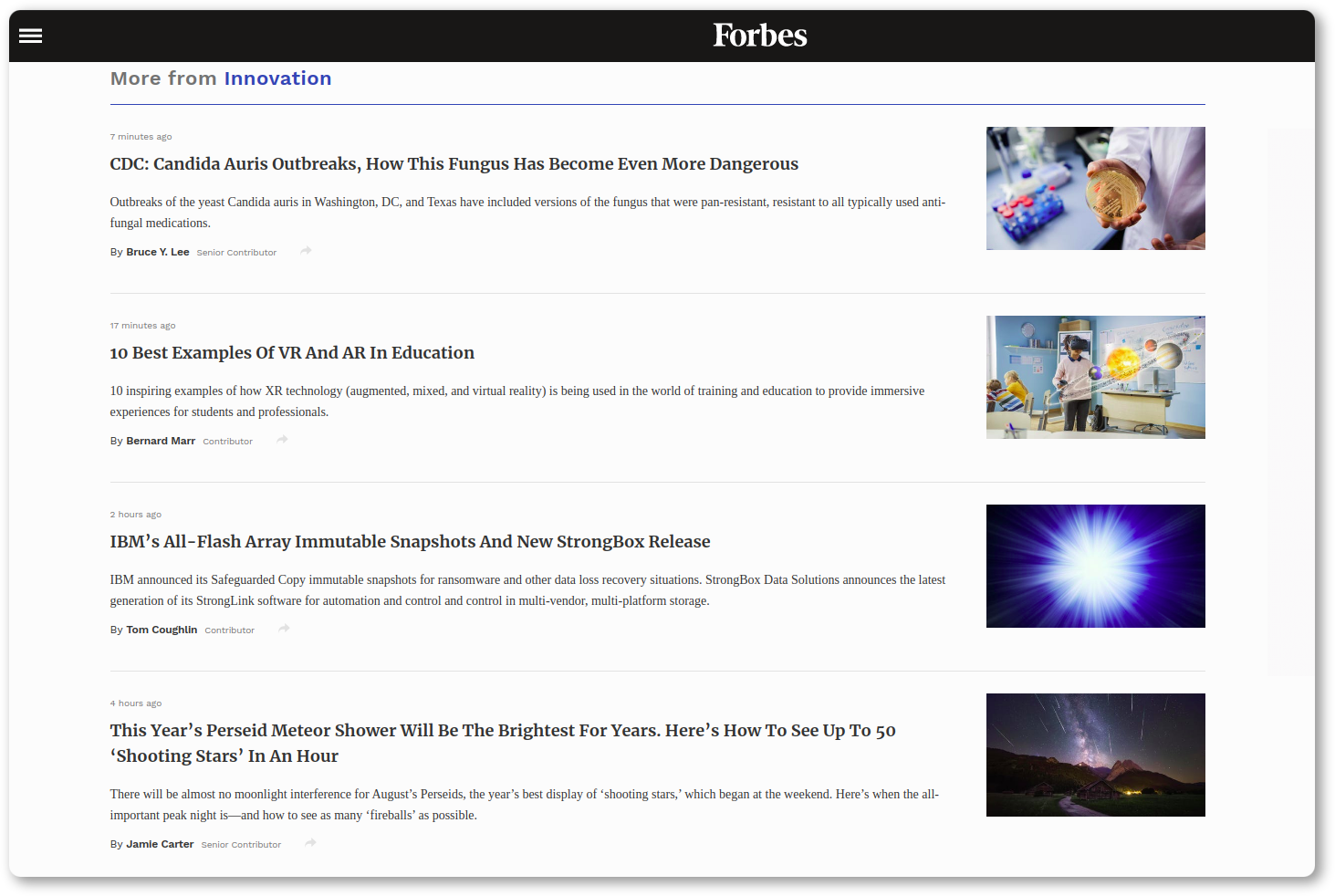This screen capture from the Forbes website features a black horizontal banner stretching from left to right. In the upper left corner, there are three horizontal lines stacked atop one another, commonly indicative of a menu icon. Centrally placed, in white lettering, is the iconic "Forbes" branding. Beneath this, in the upper left corner, bolded gray letters read "More From," followed by the word "Innovation" in blue, which is likely a hyperlink. Underneath "Innovation" is a thin blue line.

The first article headline, bolded, states, "Seven minutes ago: CDC Candida Auris Outbreaks: How This Fungus Has Become Even More Dangerous." On the right side of this headline is an image of a scientist's chest area holding a Petri dish presumably containing the fungus. The article is authored by Bruce Y. Lee.

The second section, marked by a thin light gray line, features an article posted "17 minutes ago." The bolded headline reads, "Tests: 10 Best Examples of VR and AR in Education." Accompanying this on the right side is a rectangular image depicting a teacher in a grade school classroom with an overlaid watermark-like depiction of the solar system. The article is authored by contributor Bernard Marr.

A third article is presented underneath another thin gray line, timestamped "Two hours ago." The bold headline reads, "IBM's All-Flash Array, Immutable Snapshots, and New Strongbox Release," with a dark blue image displaying a white starburst in the center adjacent to it. This piece is authored by Tom Coughlin.

Finally, the last article listed under another gray line, timestamped "Four hours ago," has a bold headline that reads, "This Year's Perseid Meteor Shower Will Be the Brightest for Years. Here's How to See up to 50 Shooting Stars in an Hour." To the right of this text is an image showcasing a night sky, featuring a meteor shower above a silhouetted hillside descending from left to right.